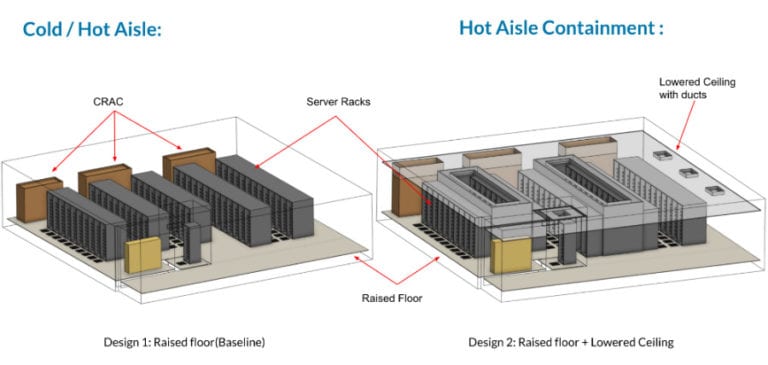The image consists of two detailed animated diagrams, each representing a distinct design for a server room, divided into two labeled sections. On the left side, labeled "Hot/Cold Aisle" in blue, is "Design 1: Raised Floor Baseline," and on the right side, labeled "Hot Aisle Containment" in blue, is "Design 2: Raised Floor and Lowered Ceiling." Both diagrams feature rows of gray server racks arranged slightly differently: while the left diagram shows rows aligned in a traditional layout, the right diagram arranges the racks more compactly, including a separate circular configuration. At the back of each setup, there are brown-colored units labeled "CRAC" (Computer Room Air Conditioners). Additionally, the right design incorporates a lowered ceiling with ducts for more efficient airflow management, illustrating a more advanced cooling strategy compared to the left design. Both designs feature a raised floor indicated at the bottom of the diagrams.